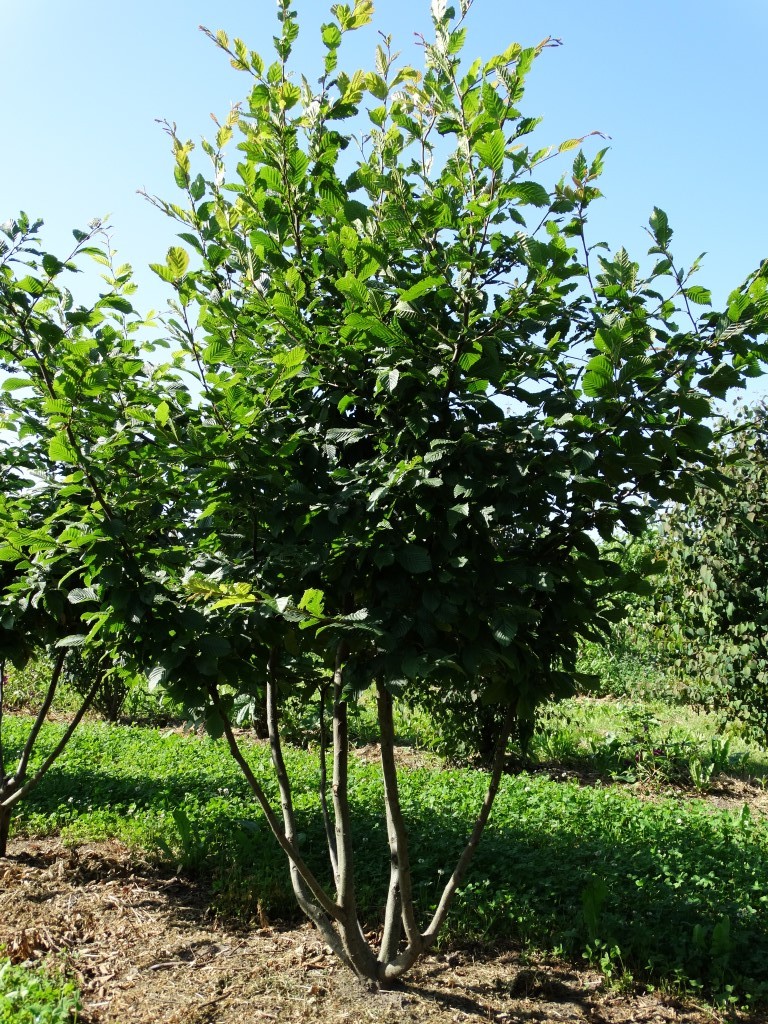This photograph captures a tall, bush-like tree set in a clearly outdoor, sunny setting. The tree, perhaps part of an orchard or an olive grove, is planted in very dry and junk-laden soil, surrounded by patchy grass and scattered twigs. The tree's distinctive wooden stems spread out from multiple roots that rise from the ground, resembling a bush at the base but transitioning into a tree with abundant green leaves about three feet up. The scene is bathed in natural sunlight under a clear, cloudless, blue sky, which enhances the visibility of multiple similarly spaced lanes of soil and additional trees in the background, adding to the structured, agricultural ambiance of the image. The overall lighting is bright, reflecting a bright, shiny day, and further emphasizes the outdoor, natural feel of the photograph.